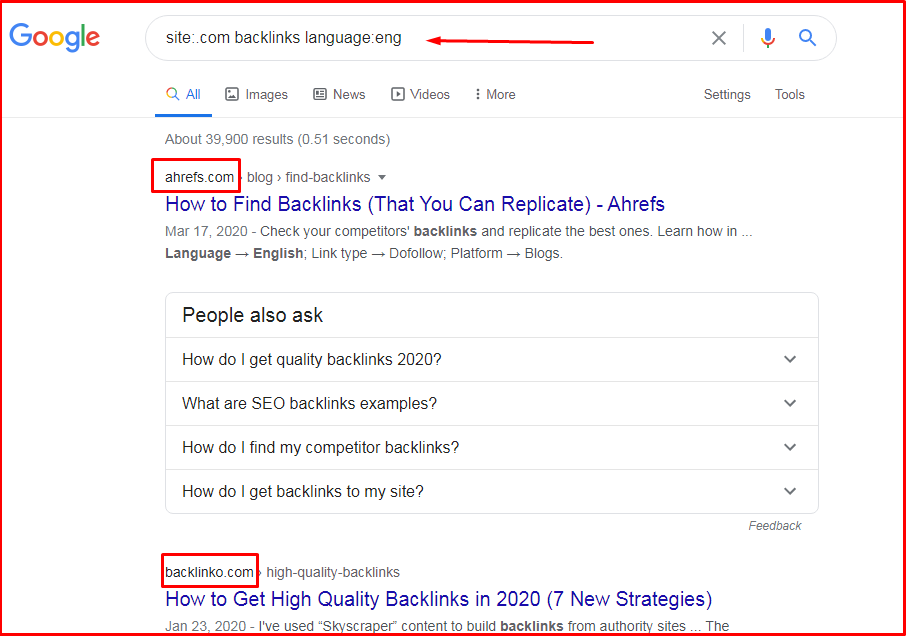A computer screen displays a Google search results page, delineated by a thin blue outline, forming a landscape-oriented rectangle. The background is predominantly white, with the complete Google logo prominently featured in the top left corner. The iconic logo comprises a capital "G" in blue, followed by lowercase letters: "o" in red, "o" in yellow, "g" in blue, "l" in green, and "e" in red.

Adjacent to the logo is a white oval search field containing the query: "site:com back links language:eng." A red arrow, pointing left, is drawn over the search field, emphasizing the typed text. To the right of the search field are the familiar symbols: an "X" for clearing the search, a microphone icon for voice search, and a magnifying glass icon for initiating the search.

Just below, there are clickable search categories; "All" is highlighted in blue and underlined, while other categories such as "Images," "News," "Videos," "More," and the options "Settings" and "Tools" are in gray with corresponding icons.

Indicating the results, the page shows "About 39,900 results (0.51 seconds)" in gray text. Beneath this, a red rectangle highlights the URL "ahrefs.com," followed by "Blog > Find Backlinks." In larger, purple letters, the result title reads "How to Find Backlinks (That You Can Replicate) - Ahrefs." Below the title, in gray, it states, "March 17, 2020," and a brief description: "Check your competitors' backlinks and replicate the best ones. Learn how in...," followed by details, such as "Language: English > Link Type: Do Follow > Platform: Blogs."

Further down, a segmented dark gray rectangle labeled "People also ask" presents additional queries: "How do I get quality backlinks 2020?", "What are SEO backlinks examples?", "How do I find my competitors' backlinks?", and "How do I get backlinks to my site?". Each query is accompanied by a downward caret, suggesting expandable answers, and the bottom section of this box includes a "Feedback" link.

Below this, another red rectangle surrounds "backlinko.com" and the text "High Quality Backlinks." The following search result title in purple reads, "How to Get High-Quality Backlinks in 2020 (7 New Strategies)."